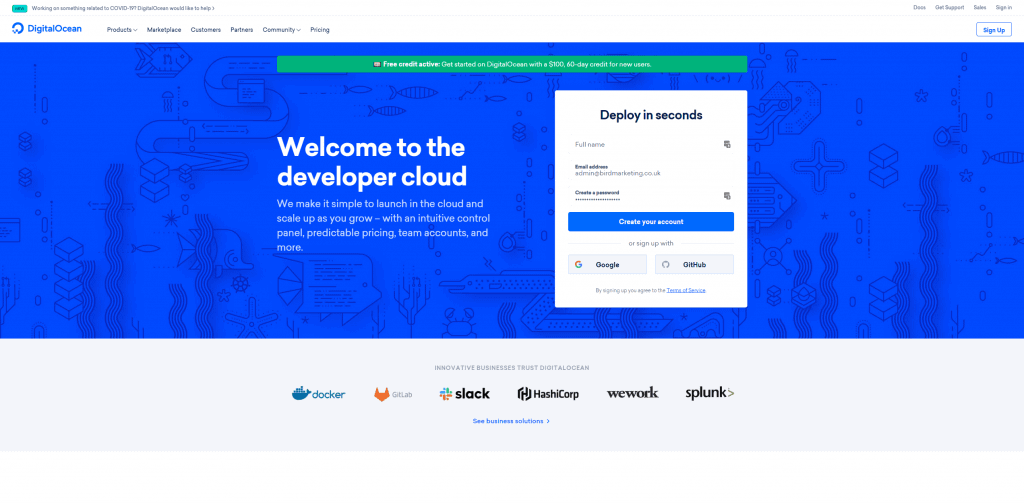The image depicts an interface with various elements, each described as follows:

At the top of the image, there is a white background featuring a baby blue button on the left-hand side. To the right of this button, there is blue text, although the exact wording is unclear due to its small size. Adjacent to this, on the far right, there is a large white space with additional blue text, including four distinct sections, though the text is illegible. 

Below this text, on the left side, there is a circular element followed by a series of six clickable items, which are black in color but similarly unclear. On the right side, there is another button, which appears to be white with blue text, set against a bluish background that features subtle scribbles. 

Centrally located within the image, there is a prominent green bar with white text written on it, though the specifics of the text cannot be discerned. Below this bar, on the left side, there is readable text stating: "Welcome to the developer cloud. We made it simple to launch in the cloud and scale up as you grow, with an intuitive control panel, predictable pricing, team accounts, and more."

On the right side, there is a white box containing black text that reads: "Deploy in seconds." Below this text, there are input fields for entering a name, email address, and password, with a blue button labeled "Create Your Account." At the bottom, there are endorsements from various places supporting the product, written in white text.